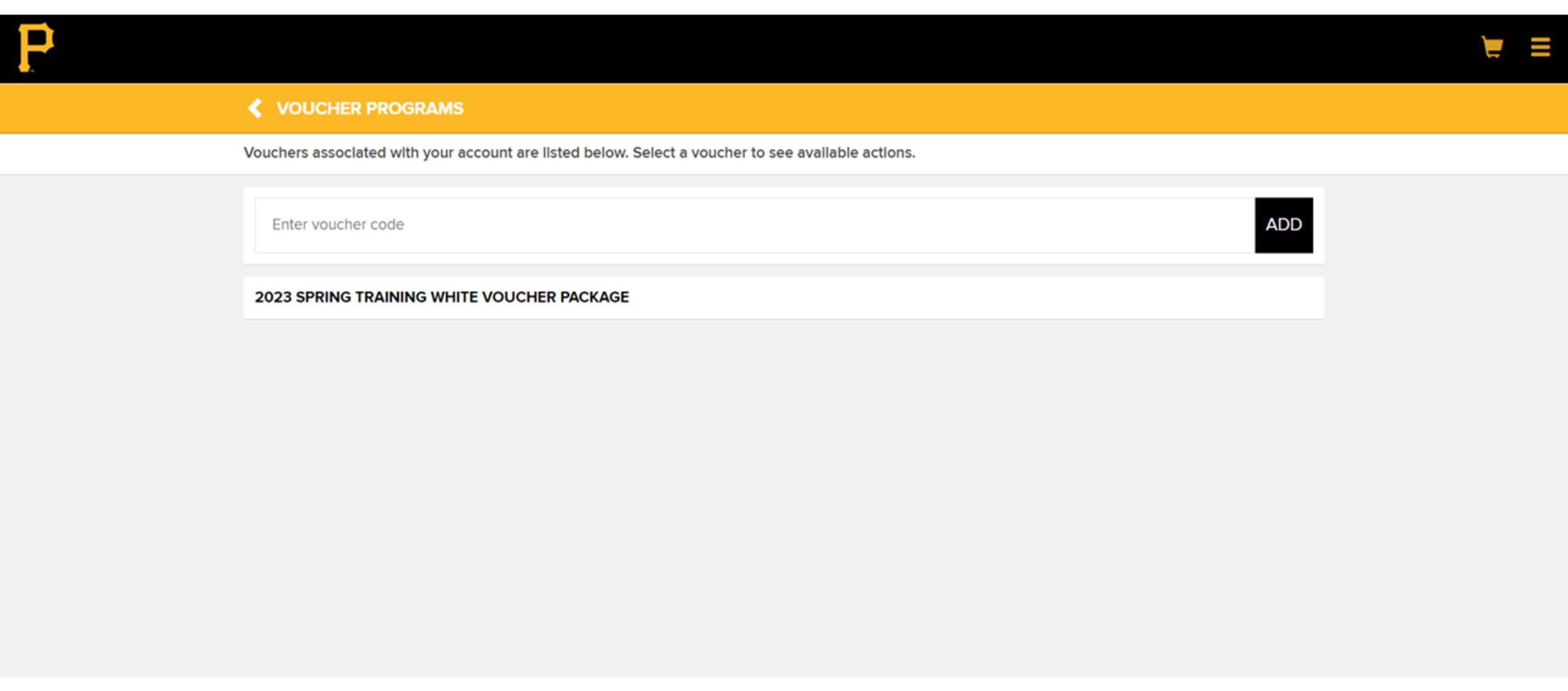This image is a screenshot of a website interface, likely related to the Pittsburgh Pirates baseball team. At the top of the image, there are two horizontal bars. The upper bar is black and approximately an inch thick, while the lower bar is a similar thickness and is colored yellow or gold. Within the yellow bar, there is a white arrow pointing back and the text "Voucher Programs" in white. 

In the top left corner of the image, there is a golden letter "P," indicating it is for the Pittsburgh Pirates. On the top right corner, there is a gold shopping cart icon, and next to it, a gold menu button represented by three horizontal lines. 

Beneath these bars, there is a white text box area that reads, "Vouchers associated with your account are listed below. Select your voucher to see available actions." Below this instructional text is a gray box, which contains a white input box labeled "Enter Voucher Code" with a black "Add" button to its right.

Further down, another white box displays text in black that says "2023 Spring Training White Voucher Package." This suggests that the user is logged into their account and has purchased the Spring Training voucher package, granting them access to spring games and other related activities.